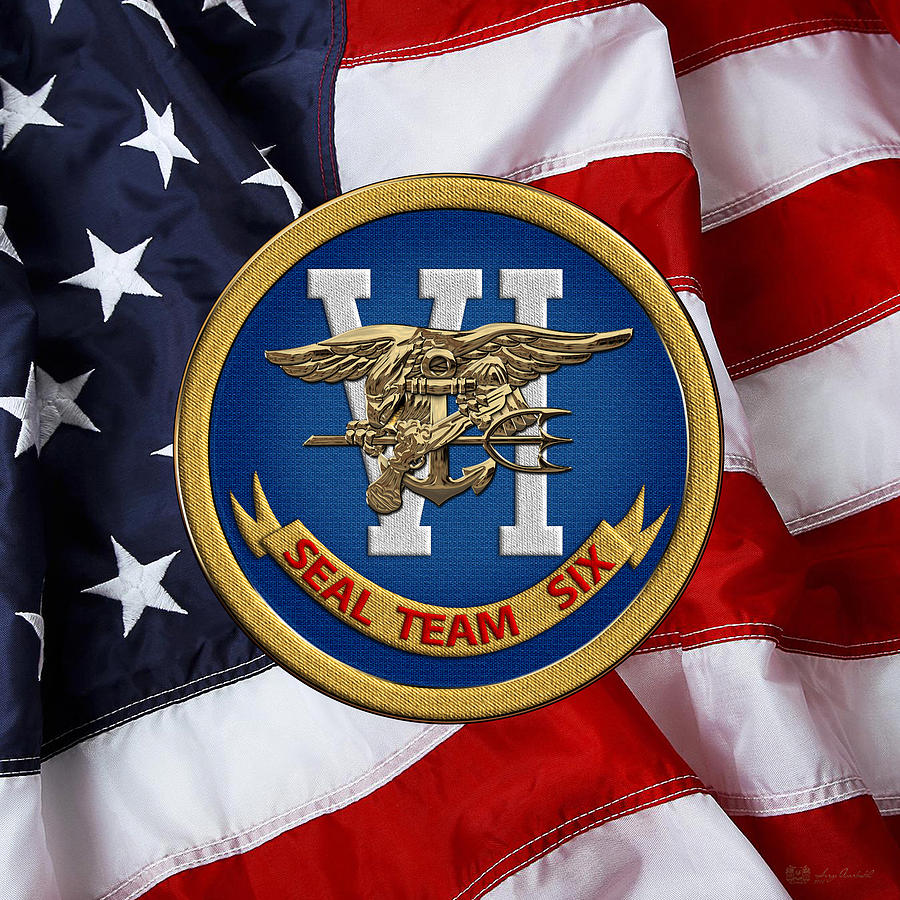This is a detailed photograph featuring a folded American flag as the background, with a prominent embossed badge centrally overlaid. The flag's distinct red, white, and blue colors are vivid, showing around seven stripes and a segment of the blue field with white embroidered stars. The flag appears purposefully folded to create a dynamic, almost flowing texture.

At the center of the image sits a circular badge with a gold trim. The badge's interior is a lighter navy blue, contrasting with the flag's darker blue. Near the top of the badge, white-stitched Roman numerals "VI" (6) are prominently displayed. Above this, a golden emblem depicting a headless bird holding three items: an anchor positioned vertically, a trident (similar to Poseidon's) oriented horizontally with three prongs pointing right, and what looks like a revolver.

Below the "VI" numeral, a gold ribbon with red capitalized text reads "SEAL TEAM 6." The detailed elements of the badge and its intricate gold-colored designs stand out sharply against the patriotic backdrop, illustrating an emblem of the elite Navy SEAL Team 6.